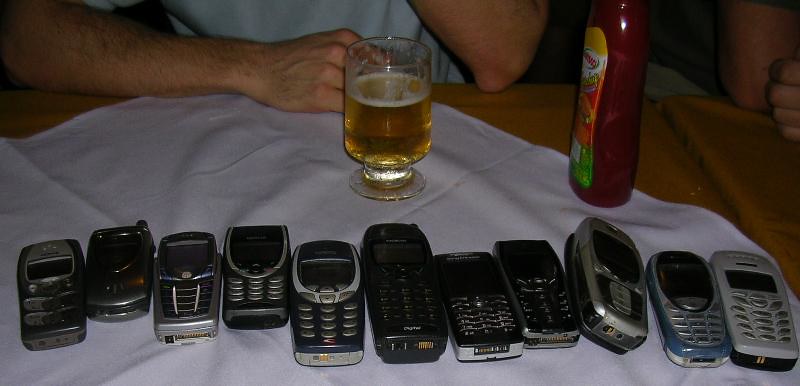In a dimly lit room casting deep shadows, two people sit at a table covered with a beige tablecloth topped by a smaller white cloth. One person is partially visible, showing only their arm and torso, while the arm of another individual can be seen beside them. On the table, there is a mix of objects, including a bottle of ketchup and a glass of beer, its light brown liquid topped with a white foam.

A striking feature of the scene is a collection of eleven old cell phones from the late 1990s to early 2000s spread out on the table. The phones, reminiscent of the Nokia brand, are bulky and metallic in appearance, with a variety of colors – black, silver, blue, and white. Among the collection is one flip phone, but the rest are the iconic brick-style models with numerous buttons characteristic of that era.